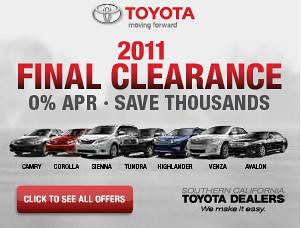The image is an advertisement for Toyota automobiles, featuring a clean, light gray and white background. At the top, the silver Toyota logo is prominently displayed, with the word "Toyota" in bold red letters next to it. Just beneath, in smaller black letters, is the slogan "Moving Forward." The main header, "2011 Final Clearance," is written in large, bold red letters. Directly below, it advertises "0% APR" and "Save Thousands" in the same eye-catching red.

Under this header, there is a lineup of seven Toyota models presented with images and names: Camry, Corolla, Sienna, Tundra, Highlander, Venza, and Avalon, each labeled accordingly beneath their respective pictures. 

In the bottom left corner, there is a red button inviting viewers to "Click to see all offers." In the bottom right corner, the text "Southern California Toyota Dealers, We Make It Easy," is displayed. The overall design is sleek and straightforward, emphasizing the clearance event and financing offers.